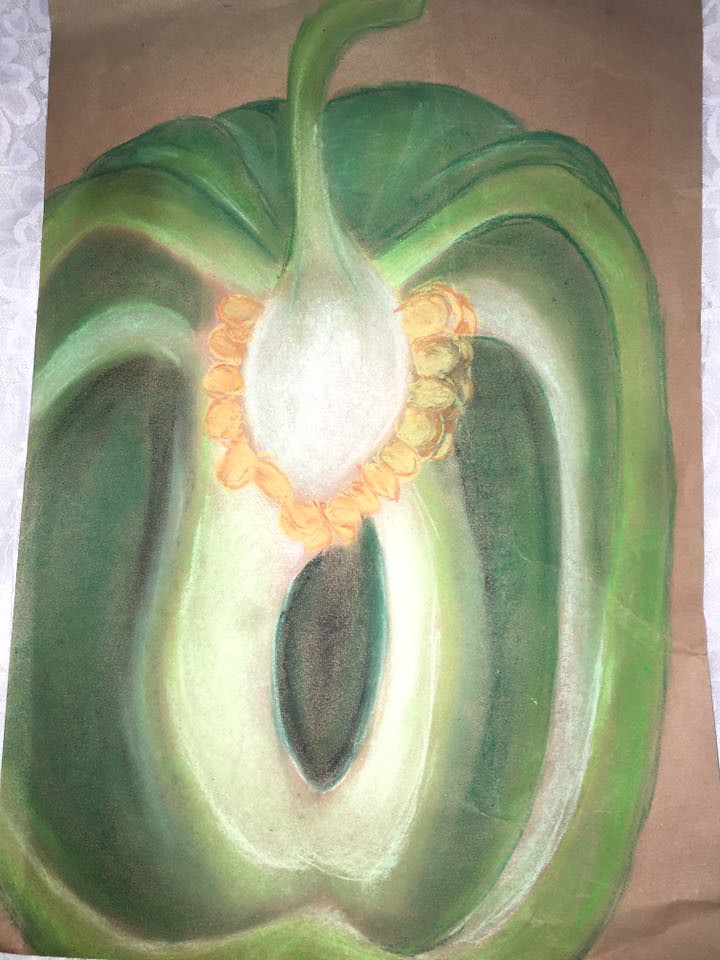The image displays a detailed illustration of a green bell pepper cut in half, revealing its intricate inner structure. The background appears to be a white and gray surface, potentially adorned with faintly drawn flowers, adding an artistic touch to the scene. The artwork itself is placed on what looks like a brown paper, suggesting either a drawing or a pastel piece, possibly even created with chalk. The bell pepper's interior showcases yellowish-orange seeds clustered around a white central bulb, which then transitions into a spectrum of green hues—from light to dark green, almost reaching a blackish-green shade in the deepest areas. The upper section of the pepper includes the white linings and a stem that gradates from yellowish-green to a darker green at the top. This composition sits atop what might be a lace tablecloth, further grounding the artwork in a domestic and delicate setting.